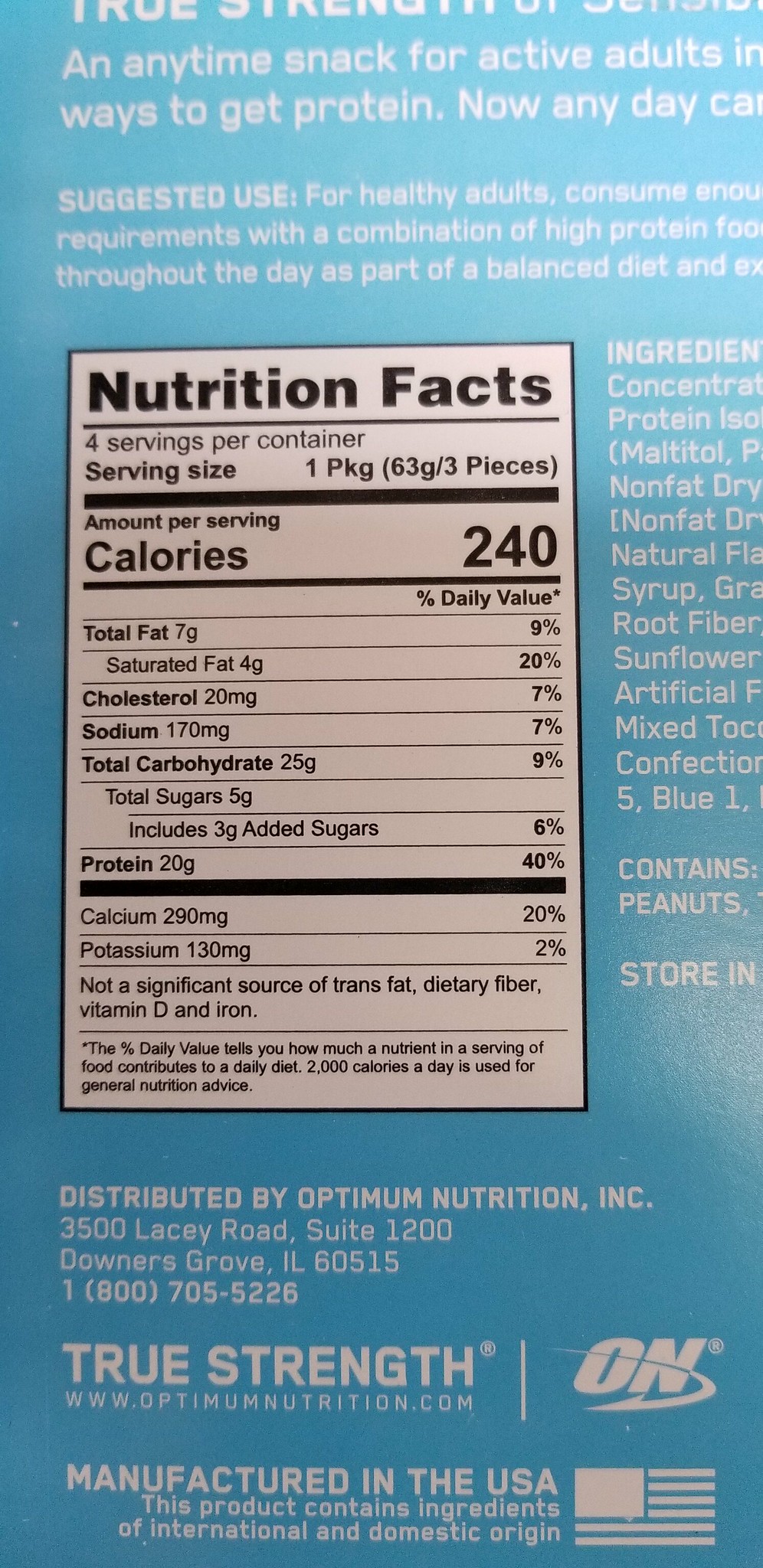The image displays the label on a product against a robin's egg blue background featuring white and black lettering. Dominating the center-left is a familiar white panel outlined in black, titled "Nutrition Facts" at the top in bold black letters. This panel reveals that the product provides 240 calories per serving, with crucial nutritional details such as 7 grams of total fat (4 grams of which are saturated fat), 20 milligrams of cholesterol, 20 grams of protein, alongside various other nutritional elements including sodium, total carbohydrates, calcium, and potassium. It's noted that the product is not a significant source of trans fat, dietary fiber, vitamin D, and iron.

On the right-hand side of the image, you can see the beginning of the ingredient panel, although only half is visible. The bottom of the label bears large white text stating "True Strength Manufactured in the USA," accompanied by a white line drawing of the American flag. Above this, it mentions the product is distributed by Optimum Nutrition, Incorporated, located at 3500 Lacey Road, Suite 1200, Downers Grove, Illinois, 60515, and provides a phone number, 1-800-705-5226.

Additionally, text towards the top of the label suggests that the product is an "Anytime snack for active adults," and outlines suggested use for healthy adults to meet their protein requirements through a diet incorporating high-protein foods. The label also contains the website "www.optimumnutrition.com" and a logo featuring the letters “ON” with a swirling arrow. Text indicates that the product contains ingredients of both international and domestic origin.